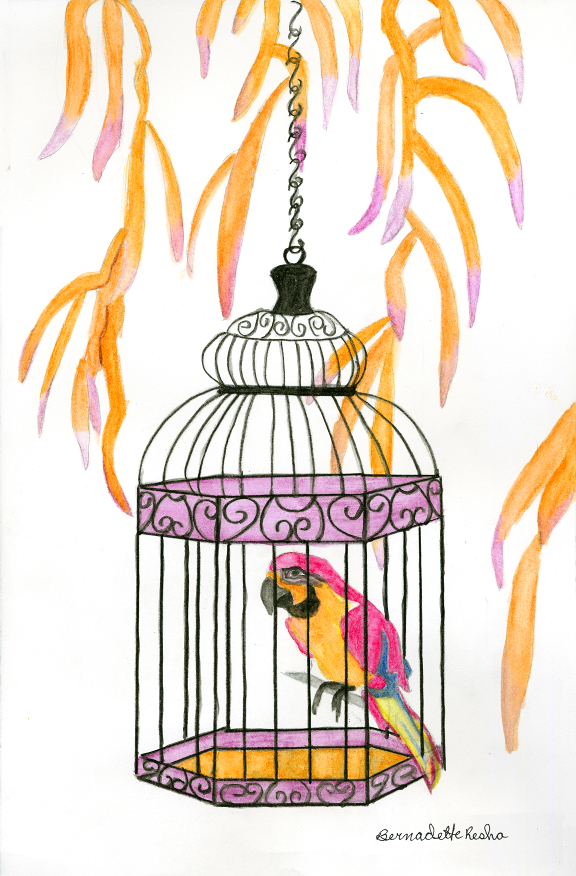This is a detailed drawing by Bernadette Resha, depicting a colorful macaw inside an ornate birdcage. The parrot features a vibrant mix of colors: an orange chest, pink feathers on its back, and touches of teal, with a black area under its chin. Its wings and body display an array of reds, blues, yellows, and blacks. The bird is positioned facing the nine o'clock direction. The birdcage itself is black and hangs from a chain, descending centrally in the composition. The cage is oval-shaped with a distinctive six-sided bottom, detailed with pink or purple trim. The entire background is a plain white, emphasizing the simplicity of the two-dimensional artwork. Above and around the cage, delicate yellow leaves with purple tips drift down, adding to the composition without overcrowding it. The leaves and the bird are rendered in translucent, solid colors, giving an almost watercolor or colored pencil effect to the image.